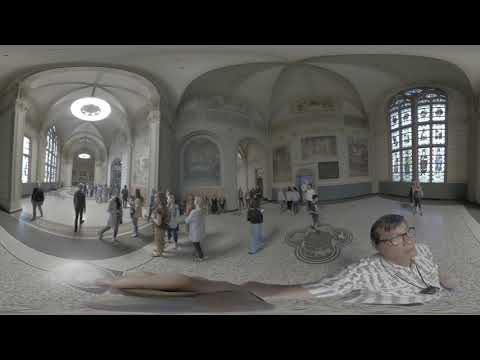The photograph captures the grand interior of a cathedral, featuring a vast, arched ceiling that exudes historical and architectural richness. A prominent stained glass window dominated by shades of blue, adorned with intricate yet indistinct decorations, is located on the distant right. The foreground features a middle-aged white man with short black hair and thick, dark-framed glasses. He wears a white and green button-up collared shirt and holds what appears to be a selfie stick or a similarly bright object, possibly reflecting light. This man is positioned in the bottom right corner, extending his hand towards the center of the frame. The marble floor beneath, mainly white with pale bluish patterns, adds to the visual depth of the scene. Scattered throughout the middle ground, roughly a dozen spectators casually explore the cathedral's splendor, walking along a hall that spans from the left to the center of the image. The overall panoramic composition, resembling a fusion of three different vantage points, captures the cathedral's ambience and the spectators' engagement in a realistic, representational style.